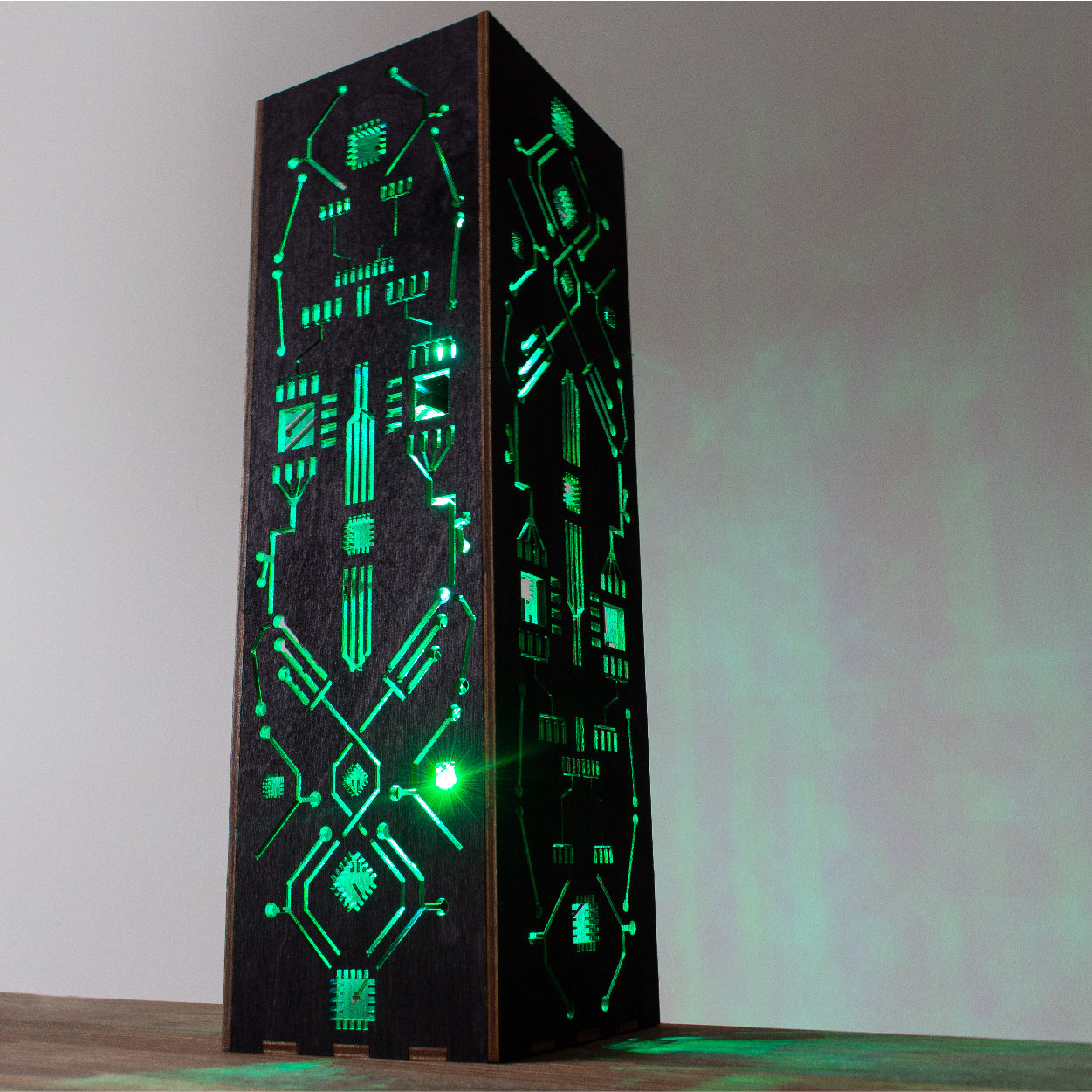This image features a tall, rectangular box standing on its end, with its length oriented vertically. Positioned against a light gray wall, the box rests on a medium-colored wooden table, supported by a small piece of wood at its base. The box, appearing to be painted black, reveals its natural wood color subtly at the corners. Viewed from an angle, the corner of the box faces the camera, allowing both the left front and right side to be visible. The surface of the box is intricately etched with designs resembling circuit board patterns, including lines, dashes, dots, and shapes that look like memory chips. These intricate designs and lines are illuminated by a vivid green light emanating from within the box, casting a greenish glow onto the table surface below. This green light accentuates the black background of the box, making the detailed etchings glow brightly against its dark surface.